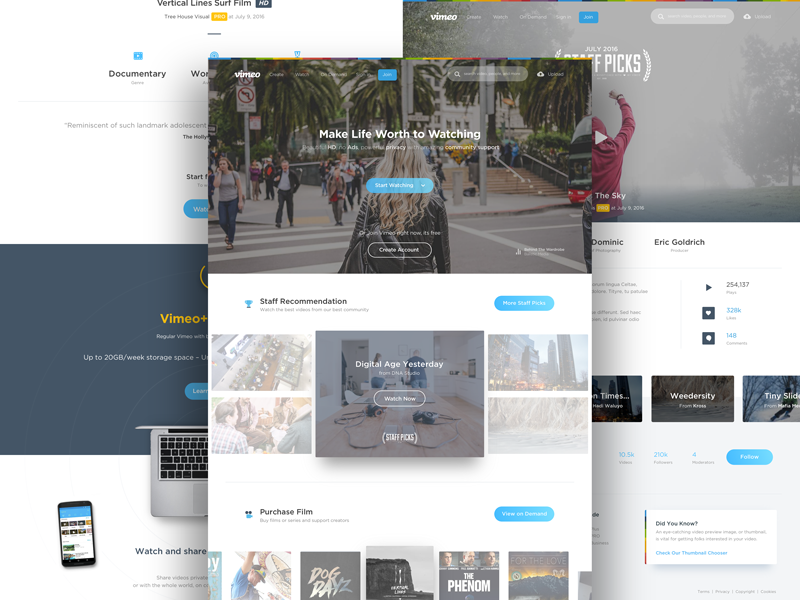The image depicts a multifaceted website interface dominated by a central pop-up featuring a prominent photograph of a woman with long blonde hair crossing a bustling street. The pop-up bears the motivating text, "Make Life Worth Watching," coupled with a distinct blue clickable button and a black one beneath it. Below this, a section with a white background displays the phrase "Digital Age Yesterday" accompanied by a "Watch Now" button. Additionally, there is a segment labeled "Staff Recommendations" and a small-print note indicating "Purchase Films" along with a clickable blue icon and thumbnail images of various films.

In the background, partially obscured by the central pop-up, are two overlapping websites. One displays the title "Vertical Line Surf Film" and mentions a documentary, although further details are hidden by the pop-up. This background also includes a gray-shaded area with orange text, illustrating a keyboard and an iPhone.

To the right of the webpage, a person in a red sweatshirt is depicted, raising their right arm. An arrow icon suggests this image is an entry point to view a video created by a name that appears as "Venmo" or "Venico." The remainder of the website presents a predominantly white background punctuated with snippets of text, images, and ends with a search bar and a "Follow" option. Additionally, there is a "Did You Know" informational box accessible for further engagement.